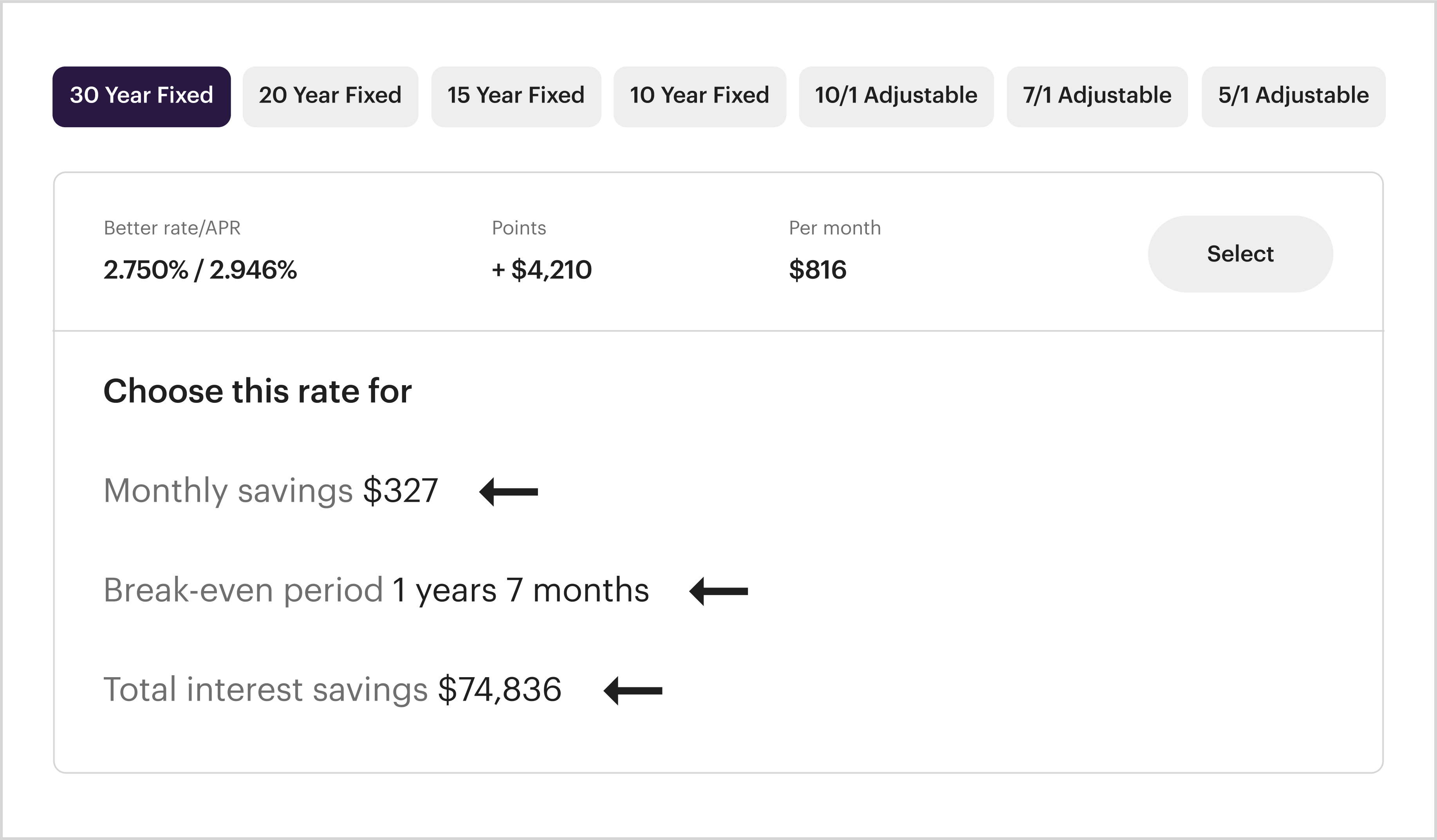The image depicts a white rectangular box with a light gray border. At the top of the box, there are seven smaller boxes arranged horizontally. The leftmost box is dark blue and has the text "30 Year Fixed" written in white. The six boxes to the right are all light gray, each containing different labels: "20 Year Fixed," "15 Year Fixed," "10 Year Fixed," "10/1 Adjustable," "7/1 Adjustable," and "5/1 Adjustable."

Below this row of boxes, a light gray horizontal line spans the width of the larger box. Below the line, there is a section with financial information starting with the text "Better Rate/APR," followed by the numbers "2.750% / 2.946%." Underneath this, it lists "Points + $4,210" and "Per Month $816."

Towards the bottom of this section, there is another light gray box with the word "Select" inside it. Beneath this box, another gray horizontal line runs from left to right. Below this line, the text reads "Choose this rate for monthly saving $327," accompanied by a left-pointing arrow.